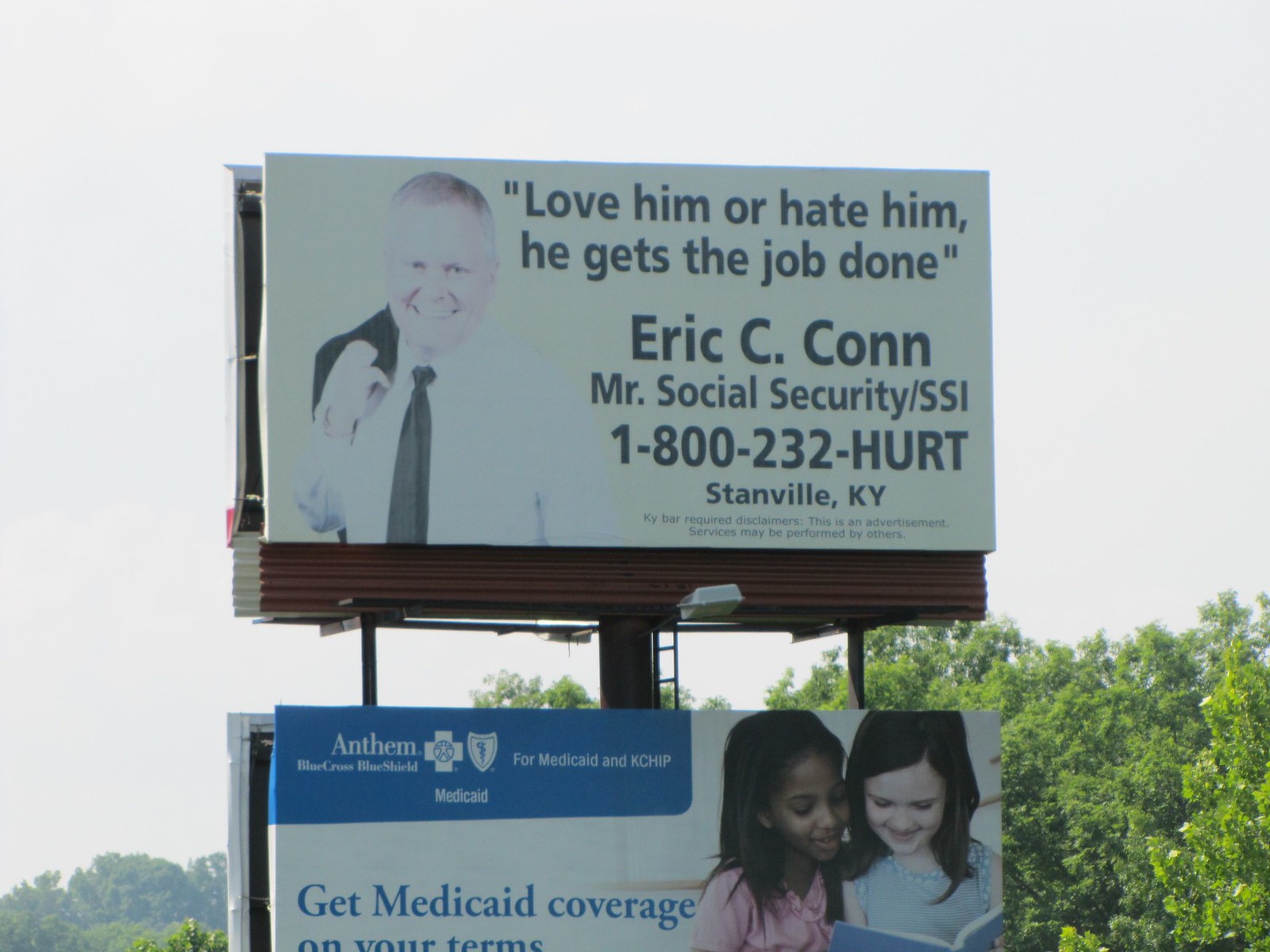This photograph captures two strategically placed billboards against a clear sky. The upper billboard features a bold message in black font: "Love him or hate him, he gets the job done. Eric C. Kahn. Mr. Social Security/SSI. 1-800-232-HURT. Stanville, KY." To the left of this text, there is a professionally taken image of a Caucasian man with gray hair, radiating confidence with a warm smile as he gazes directly at the camera. He is dressed in a white collared shirt paired with a black tie, casually holding a suit jacket over his right shoulder, projecting a no-nonsense yet approachable demeanor.

Below this billboard is another advertisement, only partially visible, promoting Anthem Blue Cross Blue Shield's Medicaid and KCHIP services. The clearly visible text reads, "Get Medicaid coverage on your terms," in blue font. Accompanying this is a heartwarming picture of two young girls, one African-American and the other Caucasian, sharing a moment of joy as they read the same book. Both girls are smiling and appear deeply engrossed in their reading, epitomizing the unity and care the Medicaid service aims to provide.